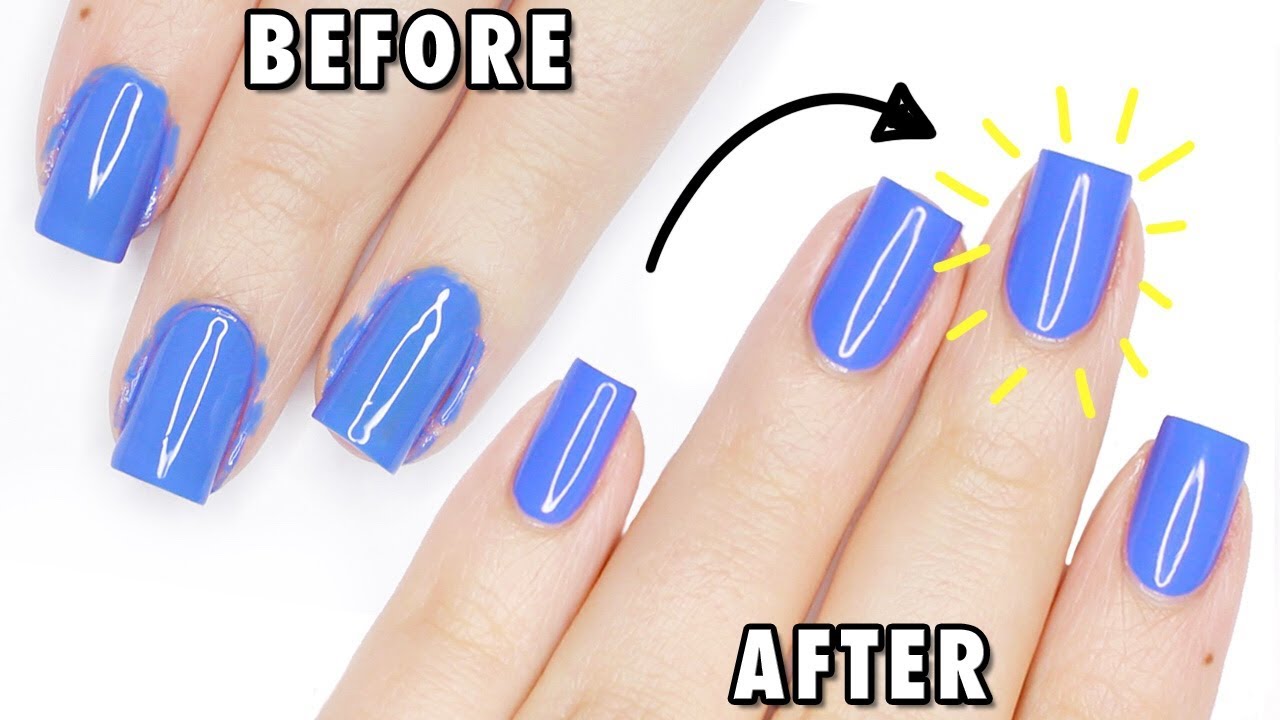This advertisement features a detailed visual comparison of a manicure's "before" and "after" conditions against a white background. On the left side of the image, three fingers with vividly blue, shiny, and bluntly-filed nails are labeled "BEFORE" in white, black-outlined letters. The polish on these nails is noticeably messy, with excess paint extending onto the surrounding skin. A black arrow directs the viewer's eye to the right side of the image, where four fingers, including a pinky, are labeled "AFTER," also in white, black-outlined letters. In this "after" view, the same vivid blue polish appears perfectly applied, neatly confined to the nails without any spillover onto the skin. The central nail is highlighted with yellow lines radiating outward, emphasizing the pristine quality of the manicure. Additionally, a small brown freckle is visible on the pointer finger, adding a touch of realism to the scene.